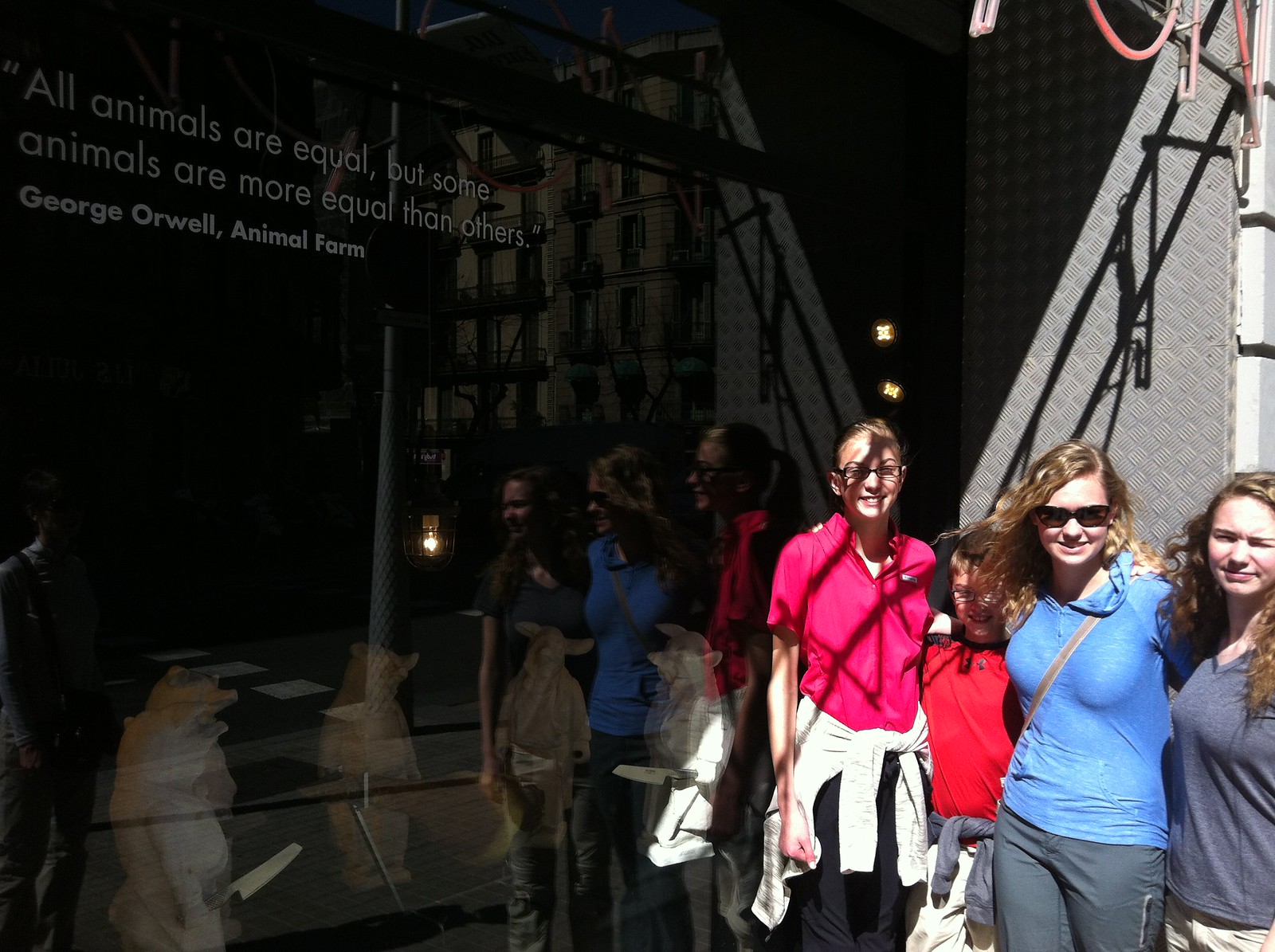The photograph captures a sunny day outside a tall building with a reflective black wall, featuring the inscribed quote: "All animals are equal, but some animals are more equal than others." — George Orwell, Animal Farm. In the lower right corner of the large frame, three women and a young boy pose, albeit poorly positioned within the composition. 

The woman on the left sports a vivid red top with a sweatshirt tied around her waist, though her features and clothing are obscured by the structure's shadows, creating black lines across her face and outfit. The young boy, standing next to her and with short hair, wears a similar red top with a gray sweater tied around his waist. In the center, a woman with long reddish blonde hair, donned in a blue top and gray pants, stands in direct sunlight wearing sunglasses. Her face glints from the sun's rays. To her left, at the very edge of the frame, is the third woman, sporting a gray v-neck t-shirt, with shoulder-length reddish-brown hair, squinting against the sunlight without sunglasses. 

All the women appear to be in their early twenties, potentially teenagers, smiling as they pose. Behind them is a gray brick facade that constitutes only a small portion of the photo, contributing to the poorly framed composition. The building's reflective glass slightly reveals indistinct sculpted figures, hinting at a potential museum exhibit dedicated to George Orwell, despite the overall darkness that engulfs a majority of the image, making the environment hard to discern.